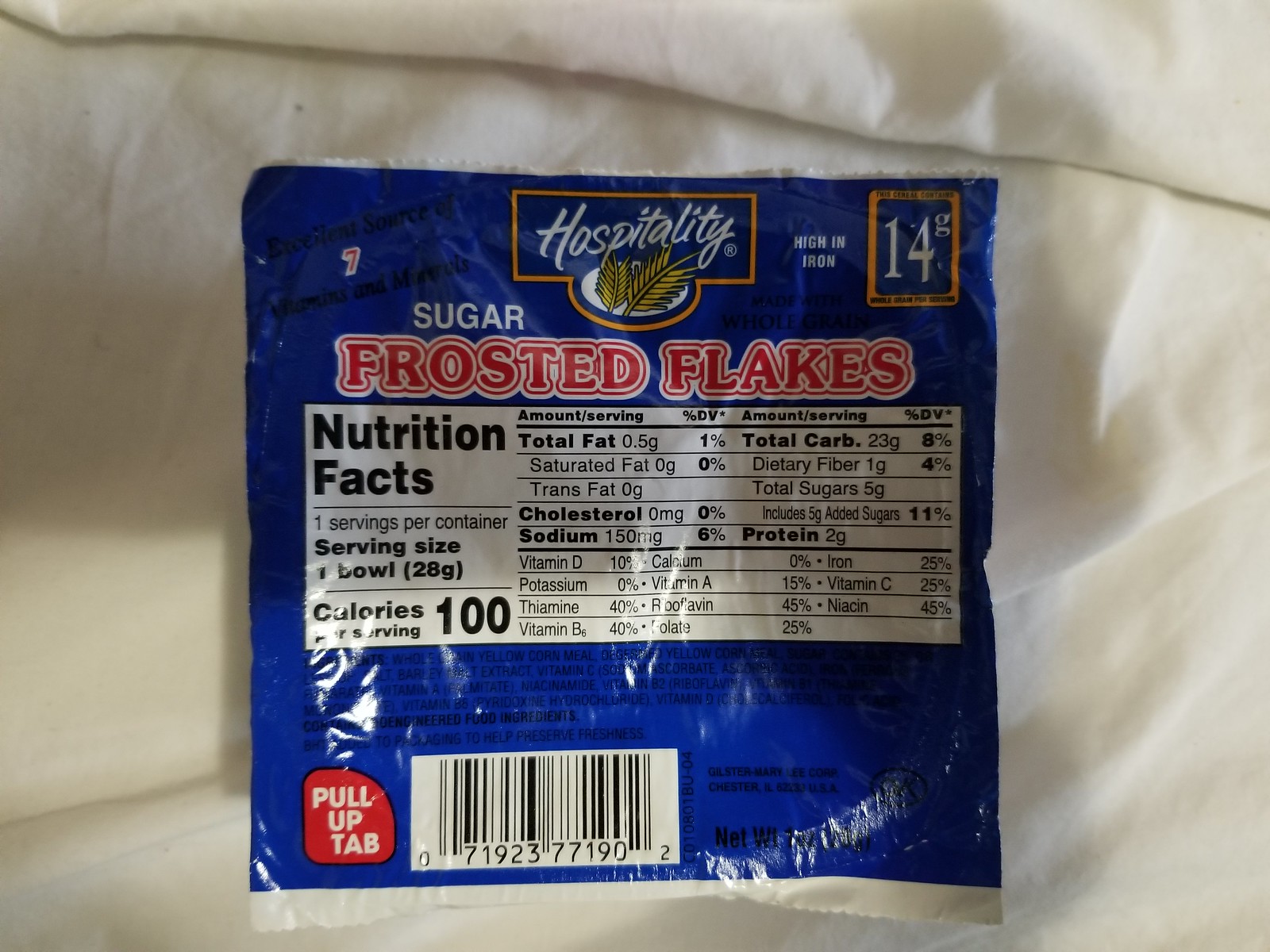The image displays a food package for "Sugar Frosted Flakes" by the brand Hospitality. The package, predominantly blue with a white and red color scheme, features bold red lettering for "Frosted Flakes" and white text for "Hospitality," which is accompanied by an image of two yellow wheat stalks. Above the product name, it states "High in Iron" with a yellow box highlighting "14 grams." The nutritional information detailed on the package includes serving size (one bowl, 28 grams), calories (100 per serving), total fat (0.5 grams), sodium (150 milligrams), total carbohydrates (23 grams), dietary fiber (4%), total sugars (5 grams), protein (2 grams), and other vitamins and minerals. At the bottom left of the packaging, a red tab indicates "pull-up tab," and nearby is a UPC code. The package itself sits on a white sheet, and a slight reflection is visible on the plastic covering.